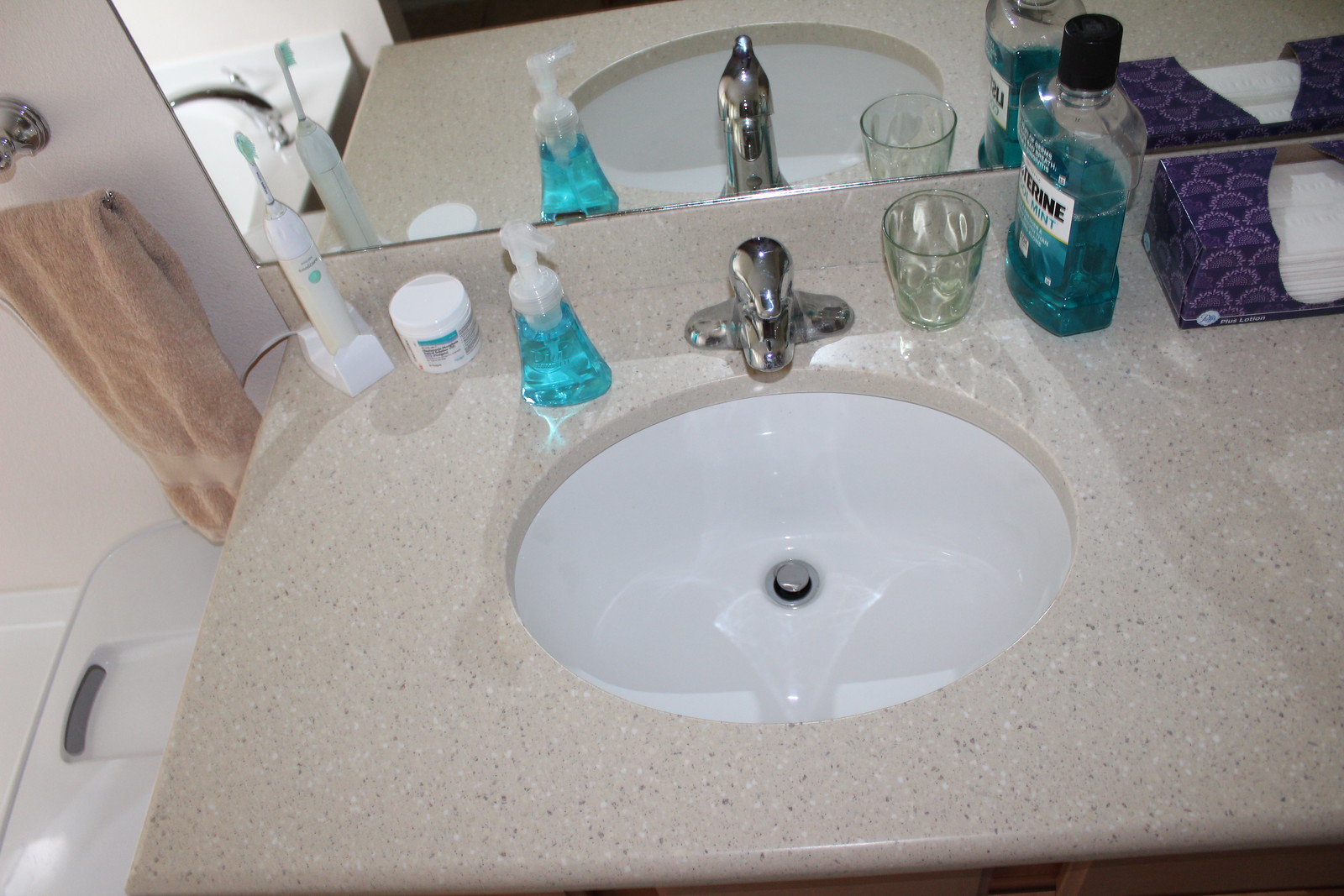The image features a rectangular sink integrated into a speckled countertop, which is cream-colored with black and white flecks. On the wall above the sink is a mirror. The sink itself has a deep, white basin with a smaller circular drain in the center. A modern faucet is mounted on the countertop above the sink.

To the right of the sink, a peach-colored towel is visible alongside the top of a trash can. The countertop hosts several items: a drinking cup, a transparent bottle of blue Listerine with a black cap, and an open purple tissue box revealing white tissues, positioned on the right side of the faucet. On the left side, there is a triangular clear bottle of blue soap and a small cylindrical jar with blue labeling. Additionally, an electric toothbrush with a round base and a small brush head is placed next to these items.